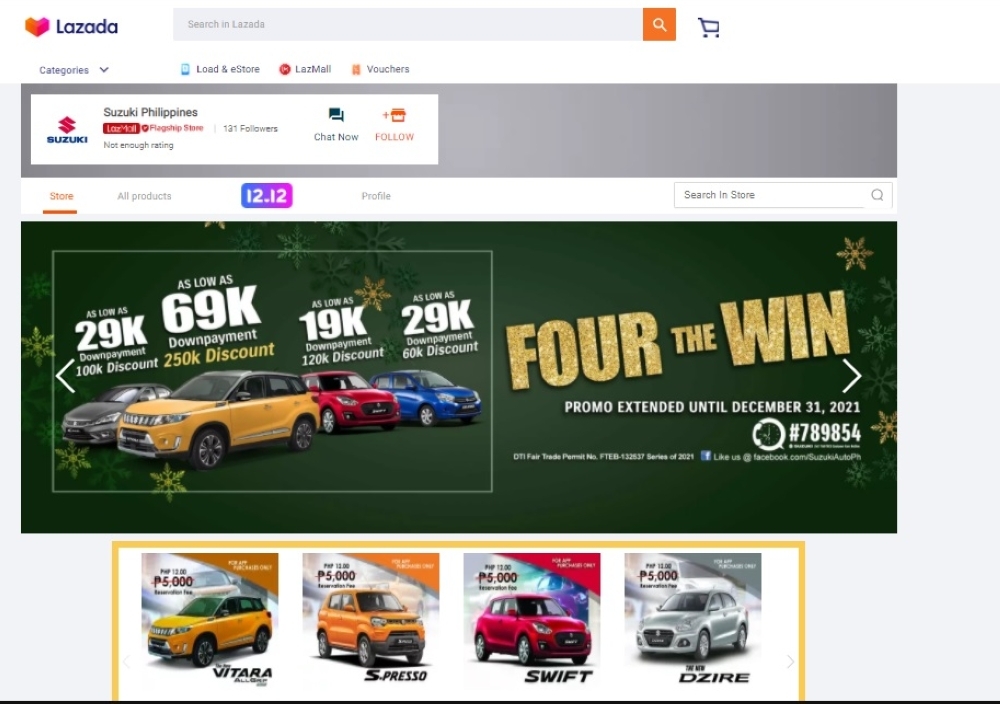The image showcases Suzuki Philippines. Prominently displayed on the left is the Suzuki emblem. Below the "Suzuki Philippines" text, there is some additional writing in red and black, though it is illegible. The account boasts 131 followers, with standard options available to "Chat Now" or "Follow". The background of the image is an olive green hue, adorned with scattered gold snowflakes, and a few more in a grayish color in the background.

The image features a boxed area displaying four Suzuki cars. Adjacent to this boxed area is the text "For the Win". Below the box is a clearer photograph of these four cars. Above the cars in the boxed area, there are numbers displayed: 29,000, 69,000, 19,000, and 29,000 respectively, likely indicating prices or some other form of numerical information. The image also notes that the promo has been extended until December 31st, 2021.